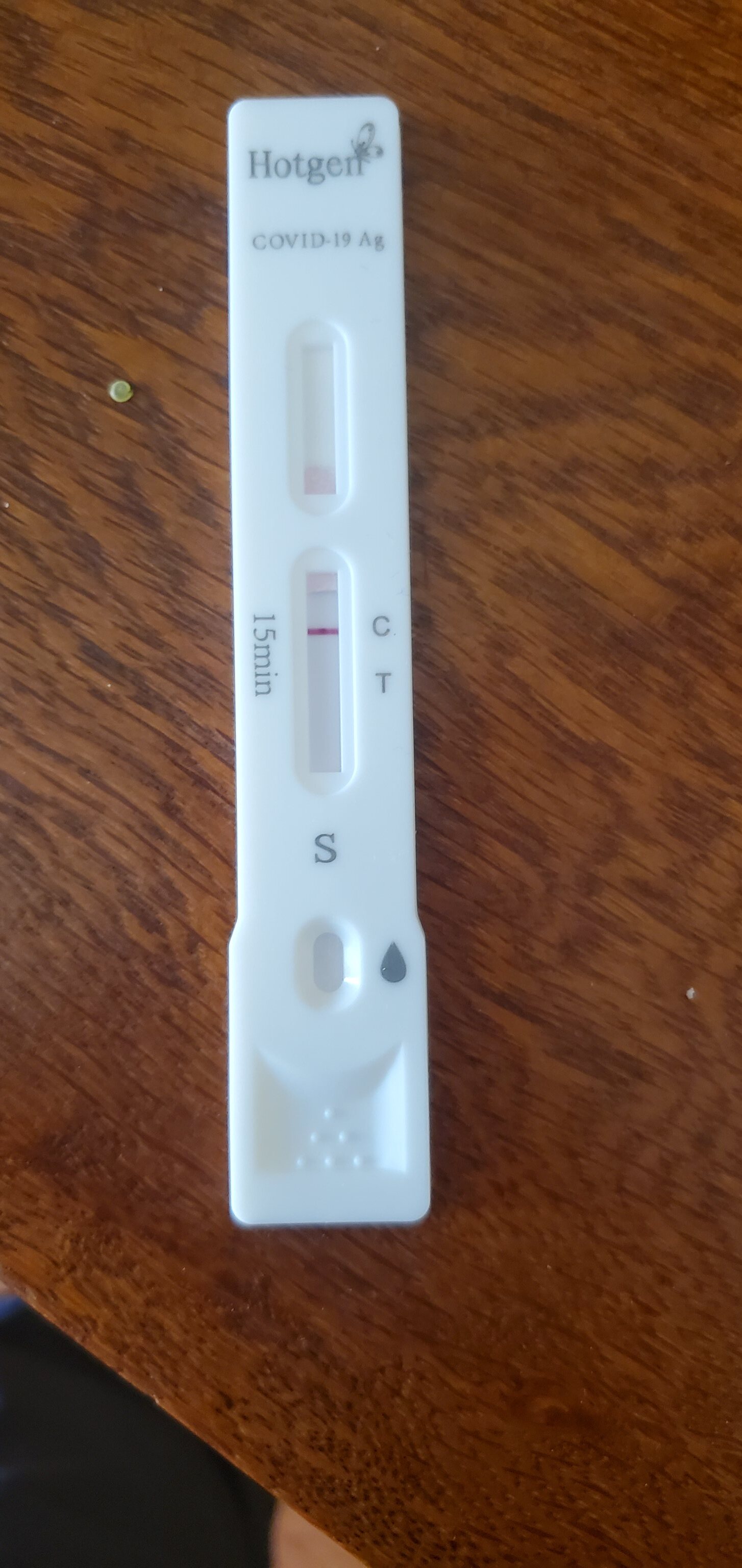A HotGen COVID-19 antigen test kit is prominently displayed on a textured wooden table. The white, rectangular strip of the test kit features a logo in the top left corner accompanied by a symbol resembling a butterfly, though not definitively clear. Below the logo, "COVID-19 AG" is clearly printed. The test strip includes a designated spot for placing a sample droplet. Further down, instructions indicate a 15-minute wait time for results, marked by the letters "C" and "T". Currently, a purple-magenta line appears on the "C" indicator, signifying the control line. The wooden table, beneath the test kit, bears visible textures and a few specks of dust and dirt, including a distinct yellow-brown mark. Notably, in the bottom left corner of the image, there is a small, triangular gap where the table surface is absent, revealing a different background.